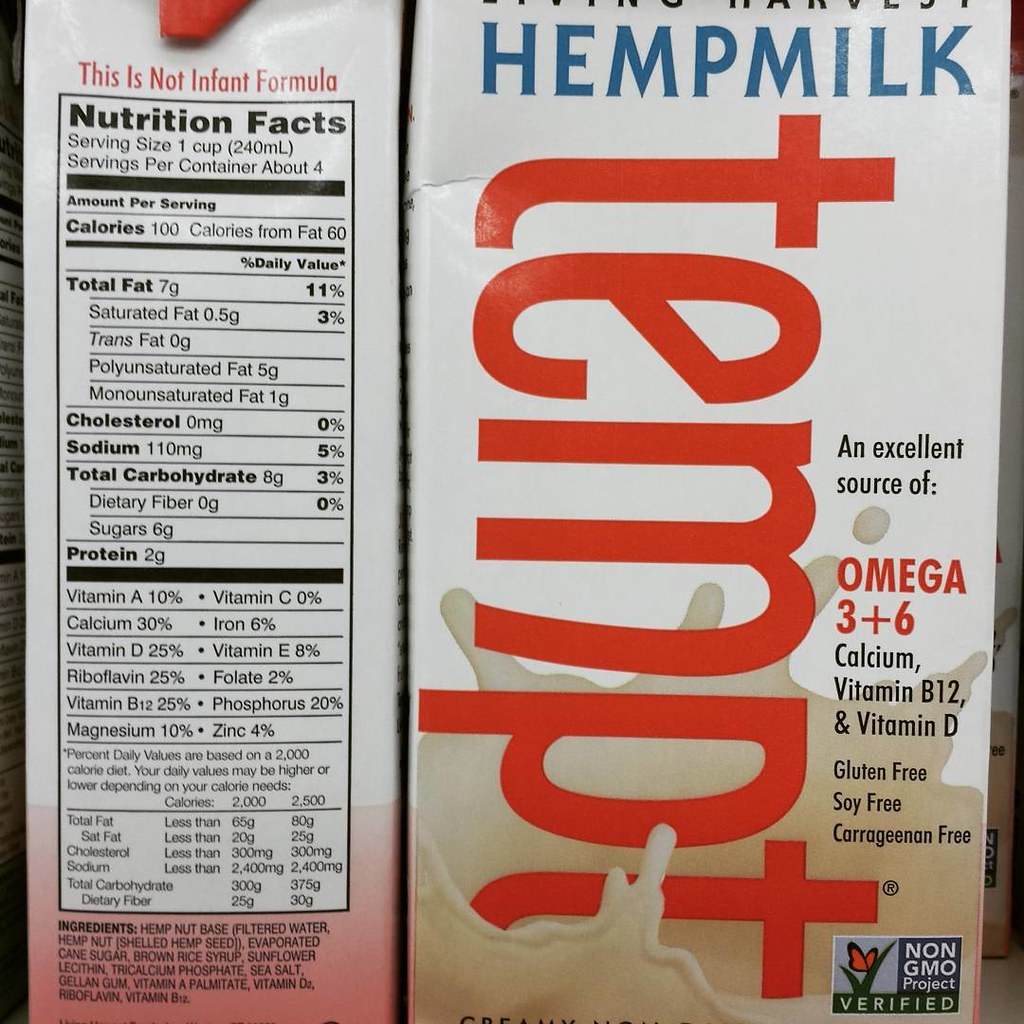This real-life photograph showcases a product labeled "Hemp Milk." The packaging is predominantly white, transitioning into a red splash at the bottom. On the right side, "HEMP MILK" is written in blue, all-uppercase serif letters. Perpendicular to this, the brand name "tempor" is displayed in large red lowercase letters, aligned vertically and partially merging into the splashing liquid imagery.

The text further details the product's nutritional benefits: "An excellent source of Omega-3 + 6" in black and red letters, followed by "Calcium, Vitamin B12, and Vitamin D" in black. Additional attributes are highlighted, including "Gluten-Free," "Soy-Free," and "No Carrageenan," alongside the "Non-GMO Project Verified" seal.

Next to the main product image is the nutritional facts panel. It clarifies that this is not infant formula, providing details such as serving size (1 cup) and a comprehensive list of ingredients: filtered water, hemp nut (shelled hemp seed), evaporated cane sugar, and brown rice syrup. The intricate design and detailed labeling aim to inform consumers about the product's health benefits and ingredients.